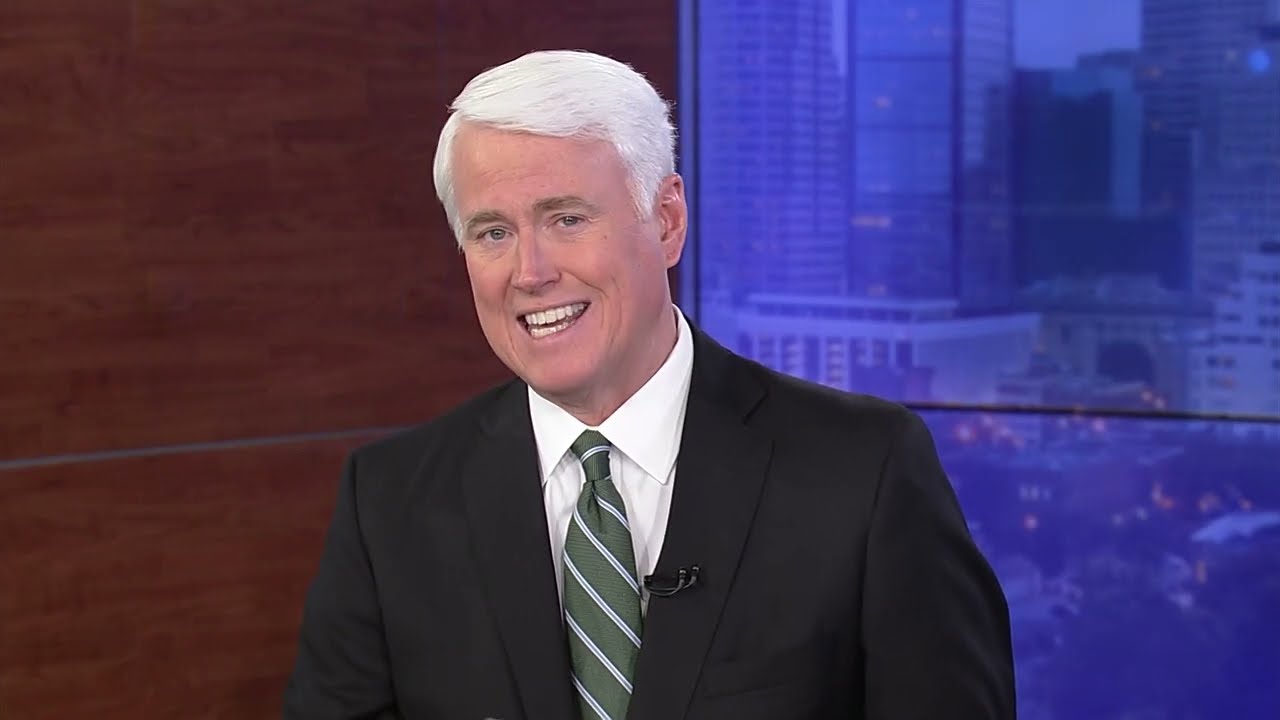The image depicts a white man, likely a news announcer, seated or standing in a high-rise news studio. He is dressed in a black suit with a white undershirt and a green tie featuring white stripes. A small microphone is pinned to the left side of his jacket’s lapel. The man, adorned with short white hair and brown eyebrows, has a slightly open mouth and appears to be speaking, with a somewhat forced smile on his face. The background includes a large window displaying a bluish cityscape to the right, suggestive of dusk, and a brownish wall on the left side. Scattered lights from the cityscape are visible, adding depth to the setting. Overall, the image captures a well-dressed announcer mid-broadcast in a modern, softly lit studio.